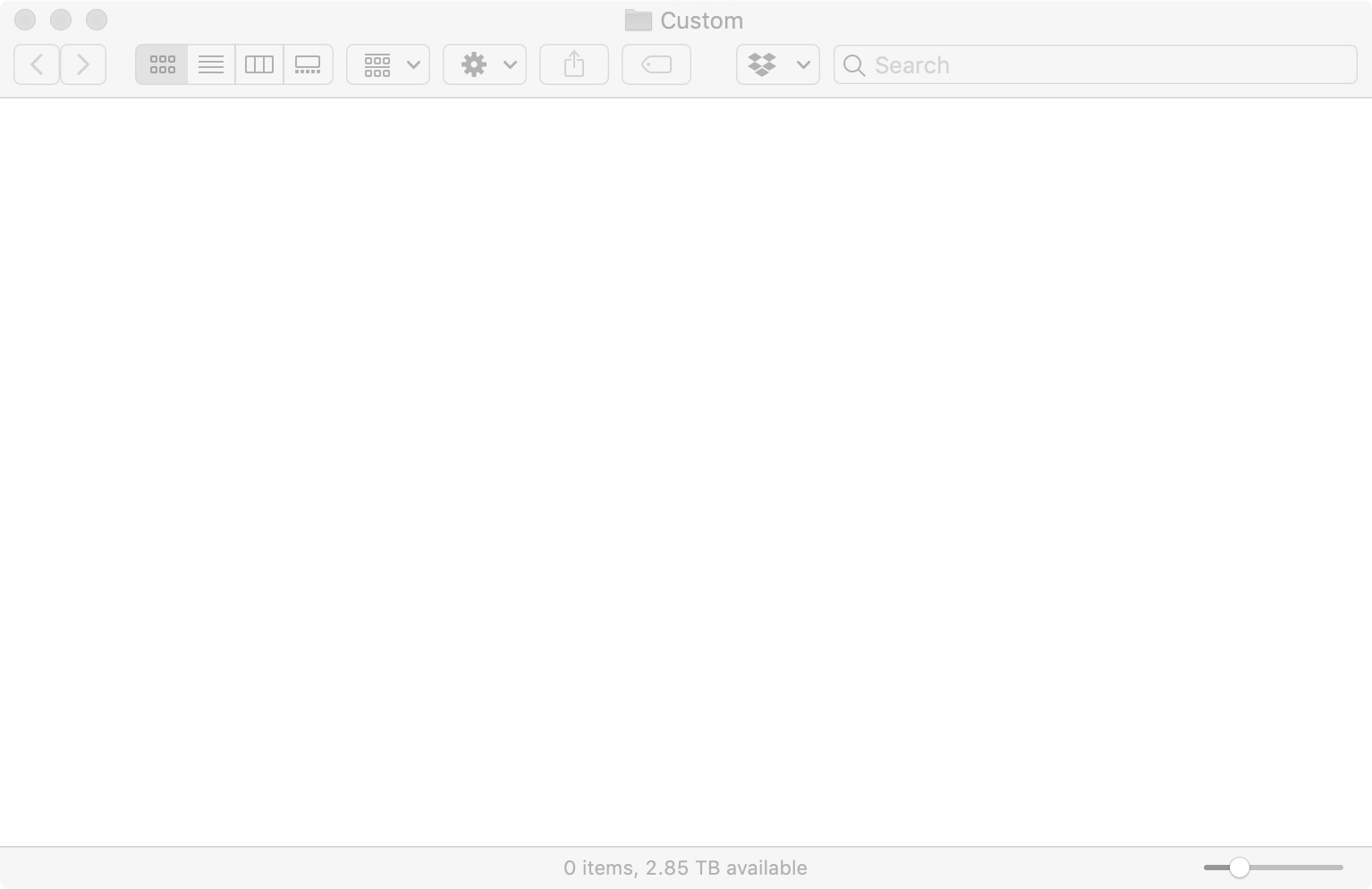The image depicts a mostly blank computer page with a distinct top section. The top portion of the page features a gray border. In the top left corner, there are three small, medium light-gray filled circles aligned horizontally. Directly beneath these circles are two square buttons: the left button has a small arrow pointing to the left, and the right button has a small arrow pointing to the right.

Next to these buttons, there's a box containing six smaller boxes arranged in two rows of three. Adjacent to this setup is another box with four horizontal lines stacked vertically. Following this, there is a box with three vertically connected bars. 

The next box contains a rectangle, beneath which there are five smaller squares. Next, there is a larger rectangular box with an intricate design: it has a line, below which are three small boxes, followed by another line with three small boxes and an arrow pointing downward.

The subsequent rectangle has a gear icon with an arrow pointing downwards. This is followed by another rectangle containing a square with an arrow pointing straight up. Next in line is a rectangle with a price tag icon inside it. Above this rectangle, the word "Custom" appears, accompanied by an icon of a folder.

Below this, on the next row, there's a rectangle containing five diamond shapes and an arrow pointing downward. Lastly, this is followed by a visible search bar with the word "Search" inscribed inside it.